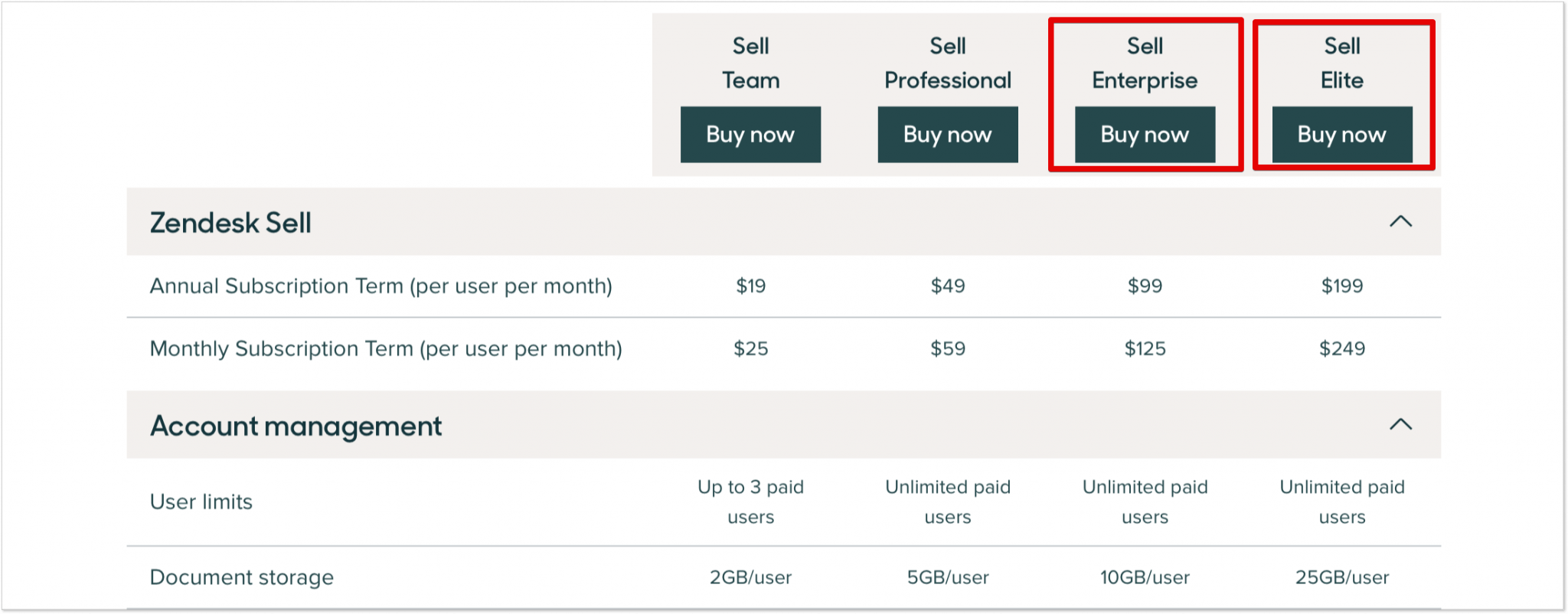The image is a screenshot of a computer display showcasing a pricing plan comparison for a software product. At the top of the screen, aligned towards the middle-right, are several boxed sections each labeled with different sales tiers. The sequence is as follows: "Sell Team" with a "Buy Now" button beneath it; "Sell Professional" with a corresponding "Buy Now" button; "Sell Enterprise" also tagged with a "Buy Now" button; and finally "Sell Elite," again accompanied by a "Buy Now" button. Notably, the "Sell Enterprise" and "Sell Elite" boxes are highlighted with red rectangles, emphasizing these specific options.

Below these boxes, on the left-hand side, the screen features the text "ZenDesk Sell" followed by "Annual subscription per user per month." This section outlines the pricing for each tier: "Sell Team" at $19, "Sell Professional" at $49, "Sell Enterprise" at $99, and "Sell Elite" at $199. The layout is structured like a comparison chart and includes sections for "Account Management," "User Limits," and "Document Storage," further detailing the features associated with each subscription level.